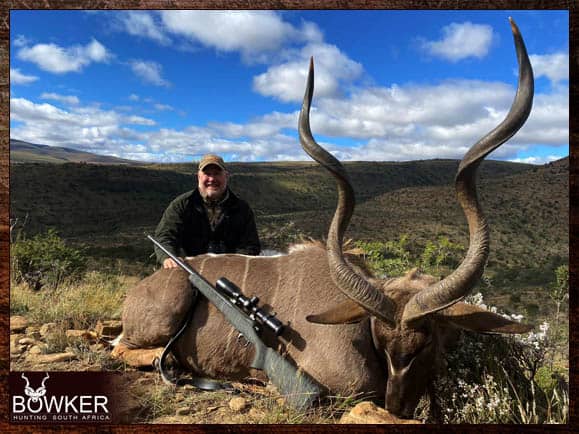This is a detailed color photograph depicting a hunter proudly posing behind a large, deceased antelope-like creature, which dominates the foreground. The animal, characterized by its light brown coat with subtle white stripes along its back, lies with its head tilted downwards, revealing long, spiraling horns that measure approximately three to four feet. The antelope's prominent horizontal ears and massive body further highlight its grandeur. Resting against the creature’s flank is a green hunting rifle equipped with a black scope, its strap trailing on the ground and the barrel pointing upwards and to the left.

Behind the majestic beast kneels the hunter, an older man with a grey beard and a broad smile. He is adorned in a green cap and a heavy jacket, possibly green or black, indicating he’s prepared for the elements. His right hand rests on the antelope's rear, a gesture of both possession and connection. The background unveils a vibrant, blue sky dotted with white clouds above a vast range of rolling hills and verdant plains, characteristic of Voldem Hill plains.

In the bottom left corner of the image, there’s white text that reads "BOKER" with a stylized animal head above the "O," followed by the phrase "Hunting South Africa," indicating the location and context of the hunt. The overall composition juxtaposes the man’s triumph with the serene beauty of the South African landscape.